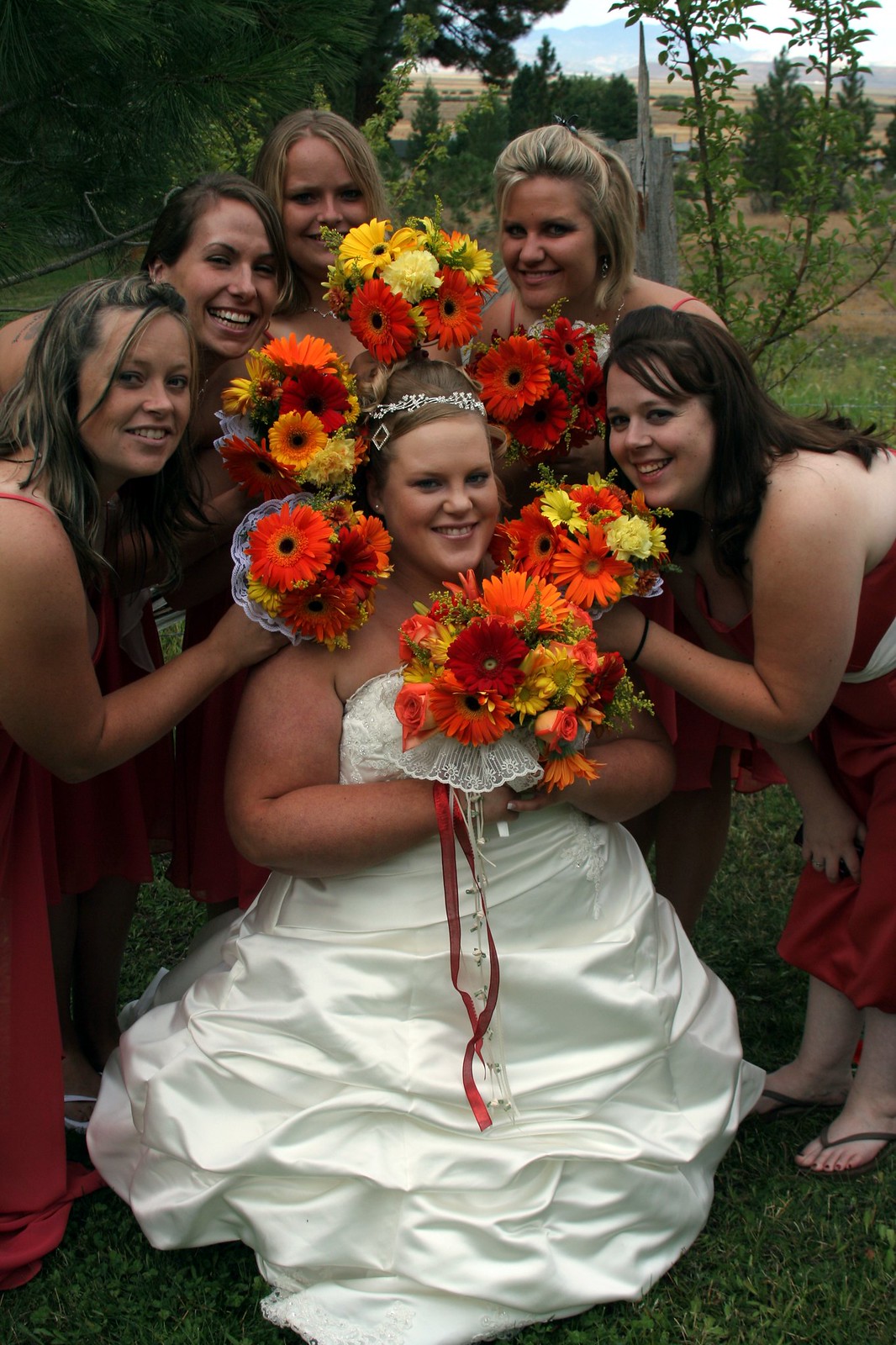In this vibrant color photograph, the bride, who appears to have just gotten married, is the focal point. She is kneeling on the ground, her legs obscured by the voluminous white wedding dress. Her attire is accentuated by a thin, silvery headdress-style band around her head. The bride holds a striking bouquet of vibrant flowers featuring orange, red, and yellow hues, including black-eyed Susans and orange roses, bound together by a rusty orangey-red ribbon cascading onto her dress.

Surrounding the bride in an arc formation are her joyous bridesmaids, each dressed in red gowns of varying lengths and designs, some strapless and others with spaghetti straps. The bridesmaids also hold similar, smaller bouquets in their hands and are smiling radiantly, their faces framed around the bride's with their bouquets positioned below their chins. The nuances of their hairstyles suggest a windy day, with some of the bridesmaids having dark brown, blonde, or light brown hair with blonde streaks fluttering gently.

The group is outside, captured amidst a lush, green garden backdrop with hills and trees in full bloom, adding to the picturesque setting. The tightly cropped image exudes happiness and anticipation, embodying the joyful essence of the wedding celebration.